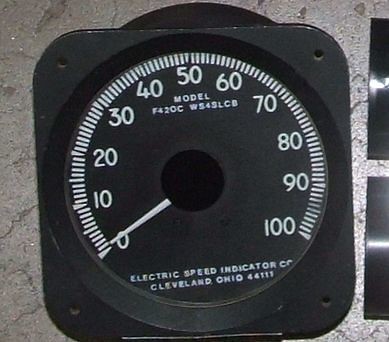This top-down photograph captures a detailed image of a speed indicator gauge positioned on a gray, possibly concrete, surface. The gauge features a standard circular shape with a scale ranging from 0 to 100, marked in white increments. At the bottom of the gauge face, the text reads "Electric Speed Indicator Co, Cleveland, Ohio, 44111." Close inspection reveals additional model information between the 40 and 60 marks, which states "Model F420CWS4SLCB."

The gauge itself has a black background with a contrasting white needle and a black center hub. The screws around its perimeter suggest it has been removed from its usual mounting location. In the background, slightly cut off on the right side of the image, are two unidentified components. The reflective glare from the camera's light source is noticeable on the gauge surface.

This image focuses exclusively on the speed indicator, which is not currently embedded in any dashboard or panel, offering a clear view of its design and features.